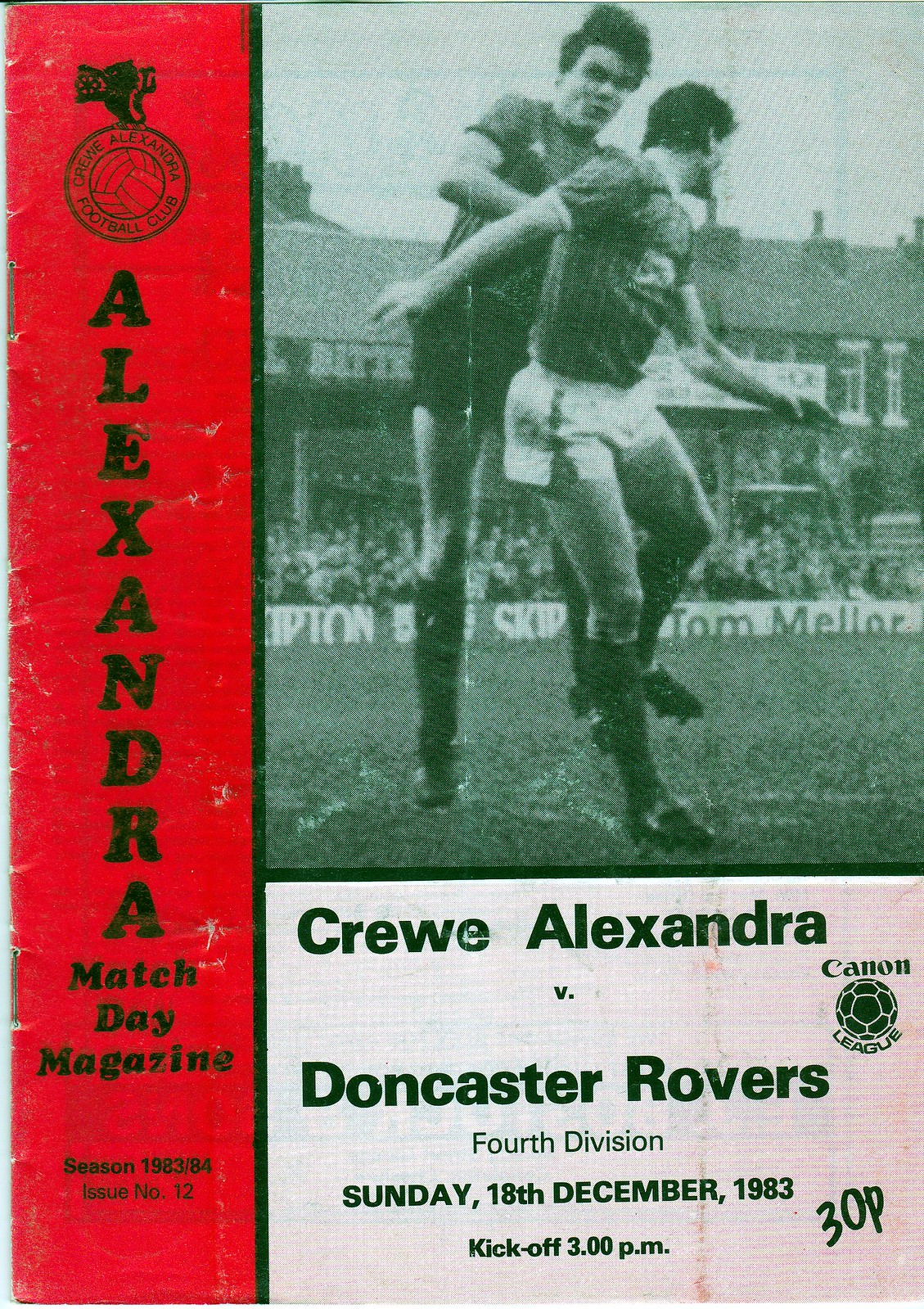The cover of the Alexandra Match Day Magazine features a black and white photograph of two soccer players in mid-action, with one man positioned behind the other as both jump into the air. Behind the players, a packed seating section is visible, adding to the sense of an energetic game day atmosphere. The top left corner of the cover showcases a circular crest with a soccer ball in the center, labeled "Crew Alexandra Football Club." Running vertically along the left-hand side is a red banner that contains the text "Alexandra Match Day Magazine, Season 1983-84, Issue Number 12." The bottom right of the magazine displays details of the match: "Crew Alexandra vs. Doncaster Rovers, Fourth Division, Sunday 18th December 1983, Kickoff 3 p.m., 30 P." The magazine cover appears very old and worn out, indicating its age and the historic nature of the event it documents.